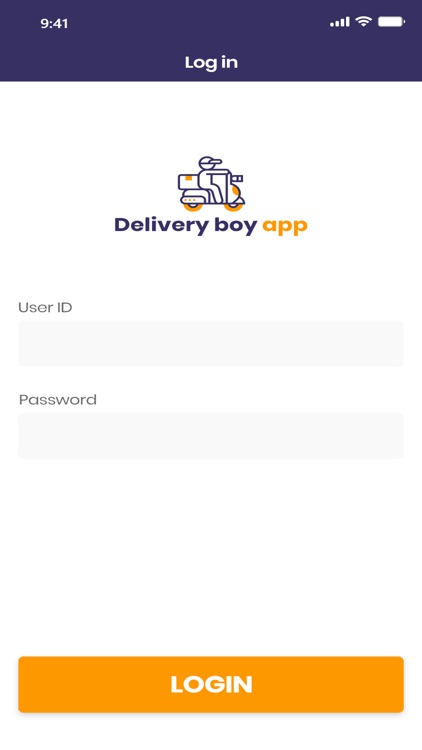The image depicts a user interface for a delivery app. At the top left corner, the time "9:41" is displayed, while the top right corner shows "1234 bars" along with Wi-Fi and battery indicators. The background is predominantly blue. The main interface features a white background with a blue border. 

Central to the image is an illustration of a person wearing a hat, sitting on a scooter. The scooter is colorfully painted, signifying the delivery service. The text "Delivery Boy App" is prominently displayed.

Below the illustration, there are input fields labeled "User ID" and "Password." An orange rectangle with white text in the center reads "Login," inviting users to access the application.